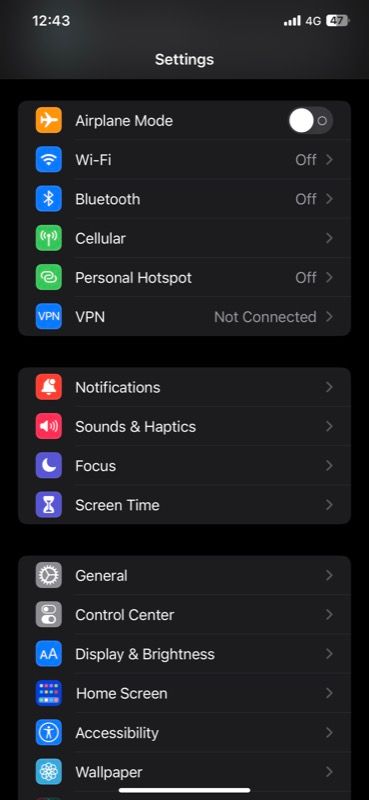This screenshot is captured from a cell phone and displays the device's settings page. The image is vertical and rectangular with a dark gray or black background. 

At the top of the screen, the status bar shows the current time at 12:43, a battery icon, and a 4G network status with full signal strength (four bars). Centered at the top is the title "Settings," indicating the user is navigating the device's settings menu.

The interface is structured with three distinct sections of settings options, each listed with icons in colored boxes on the left-hand side. 

In the first section:
- The top option features an orange box with an airplane icon, indicating "Airplane Mode," which is turned off.
- Below it, a blue box with a Wi-Fi icon labeled “Wi-Fi” is shown, and the status is off.
- Next, there is a blue box with a Bluetooth symbol that looks like a ribbon or two intersecting kites, labeled “Bluetooth,” which is also turned off.
- A green box with a cellular tower icon labeled “Cellular” follows.
- The next option is personal hotspot, illustrated by a green box with two chain link icons, and it is off.

Overall, the page lists a total of three sections of settings options with six options in the first section, followed by another four in the second, and an additional six in the third, demonstrating a comprehensive selection of available settings for the user to manage.